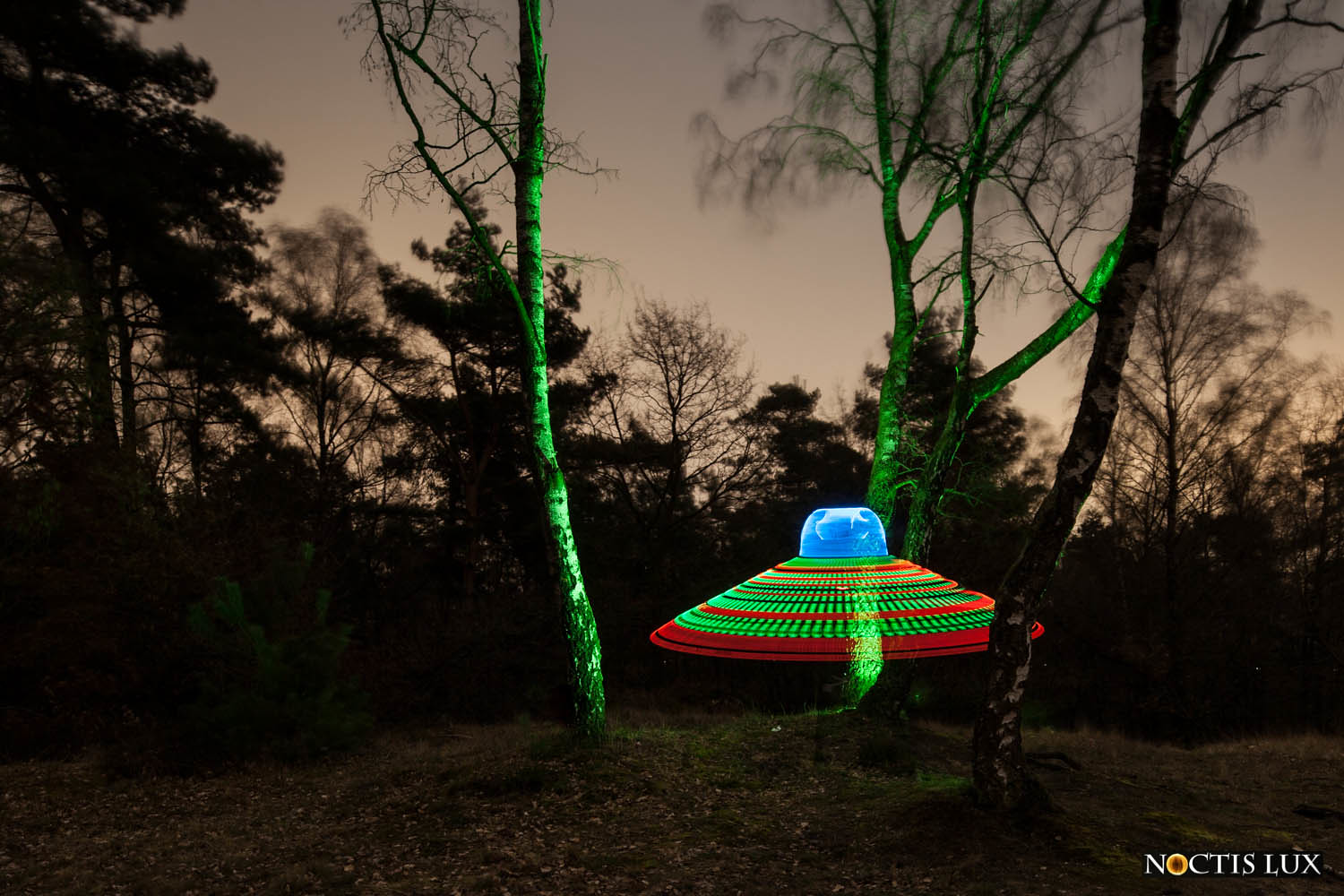In the image, a vibrant and contrasting scene is captured. The background is dominated by a dark, overcast sky and silhouetted trees, creating a somber and muted atmosphere. However, in stark contrast, the foreground features a brightly illuminated object that resembles a combination of an umbrella and a mushroom, likely serving as a lawn decoration. The top of this whimsical structure radiates a brilliant blue light, while its underside, flaring out like an umbrella, is vividly colored in red and green. This colorful object casts a mystical green glow on the surrounding trees, except for one tree directly in front, which remains dark and unaffected by the luminescence. The intense brightness of the object suggests it is powered by LED lights, adding a fantastical element to the scene. A logo is subtly positioned in the bottom right corner, possibly indicating the brand or creator of the decoration.